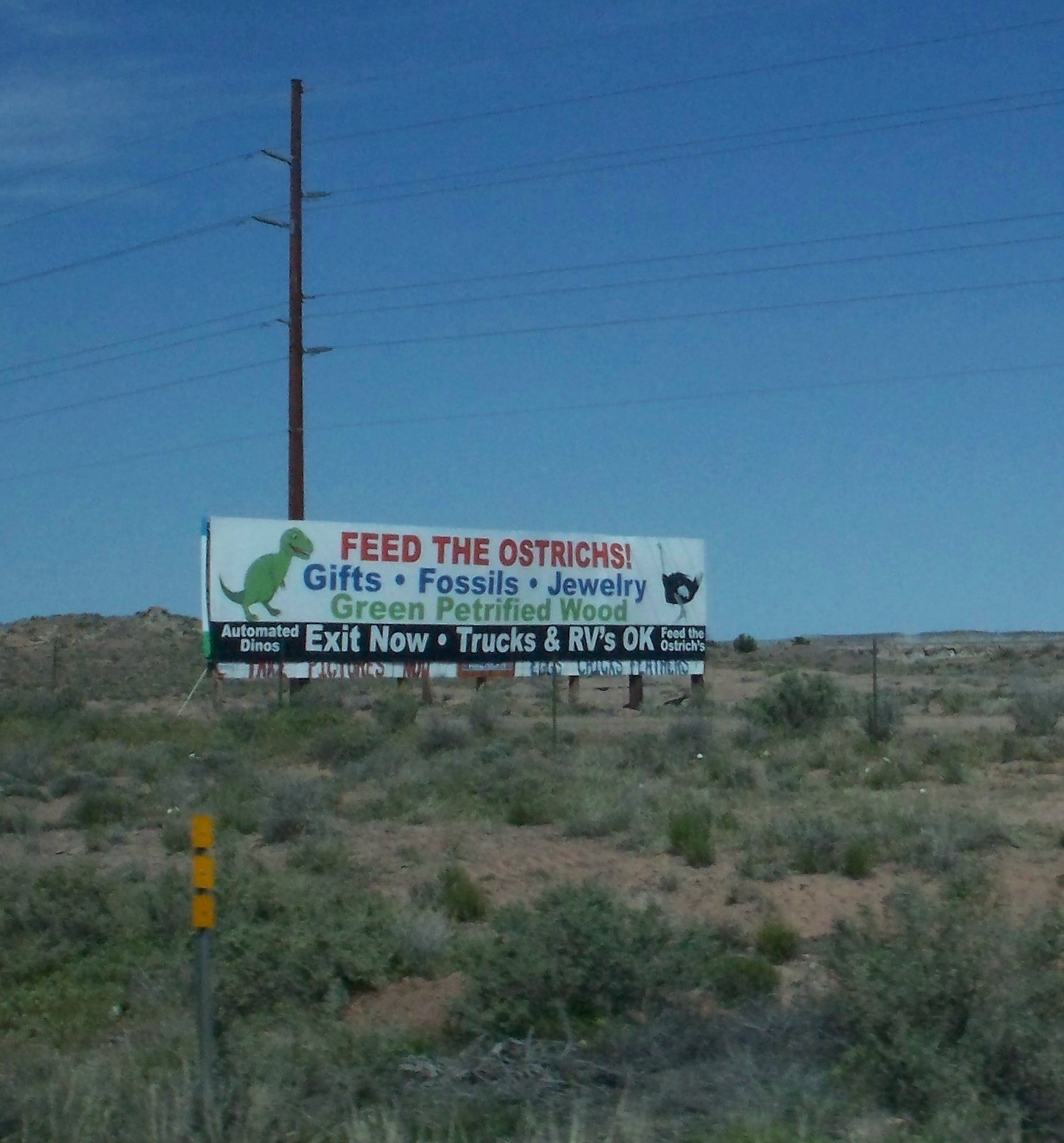The image captures a roadside scene suggestive of the Southwestern United States, characterized by a dry, sandy terrain dotted with sparse green plants, cacti, and weeds. Dominating the upper half of the photograph is a wide blue, cloudless sky, intersected by a telephone pole with multiple wires stretching horizontally across the background.

Central to the image is a white rectangular billboard located about two-thirds of the way back from the foreground. The billboard, designed to promote a roadside attraction, features various colorful texts: at the top, bold red letters with an exclamation point proclaim, "Feed the Ostriches!" Below this, in blue text, it lists "Gifts, Fossils, Jewelry," followed by "Green Petrified Wood" in green text. A black banner at the bottom of the sign announces in white letters, "Automated Dinos, Exit Now, Trucks and RVs Okay, Feed the Ostriches."

The billboard also includes vibrant illustrations: on the left side, a large black and white ostrich faces leftward, while on the right side, a green Tyrannosaurus rex faces right. Near the bottom left of the image stands a green metal rod with three yellow triangular reflectors, providing a marker for the roadway. Hills rise gently to the right, grounding this vibrant scene in its arid, desert-like setting.